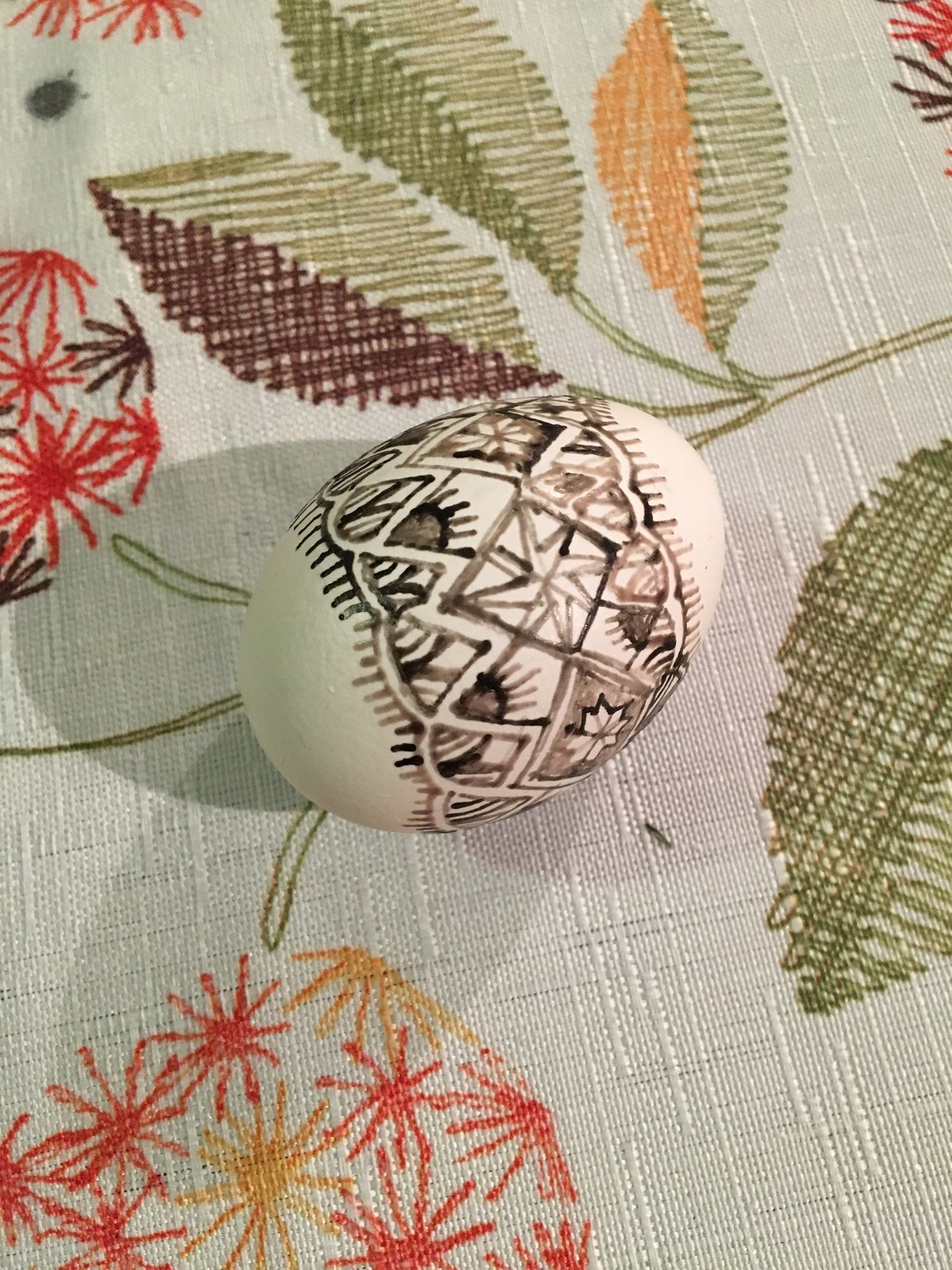In the image, there's a white egg meticulously decorated with an ornate pattern using black or brown marker. The intricate design, resembling lattice work or a fence, wraps around the center of the egg, leaving the top and bottom unpainted. The pattern is highlighted by starburst shapes and detailed triangles, indicating a significant amount of time and care was spent on its creation, potentially for an occasion like Easter.

The egg rests on a delicate white tablecloth adorned with embroidered details. The embroidery features leaves in green, orange, and brown hues, alongside red and orange flower details with visible stems, contributing to the tablecloth's intricate and delicate appearance. The fabric itself has a slightly rough texture and is covered in various designs that include ball-like shapes with red lines radiating out, reminiscent of spiders, and pale yellow-gold accents. In the background, a small black dot is visible, adding to the tableau's complexity.